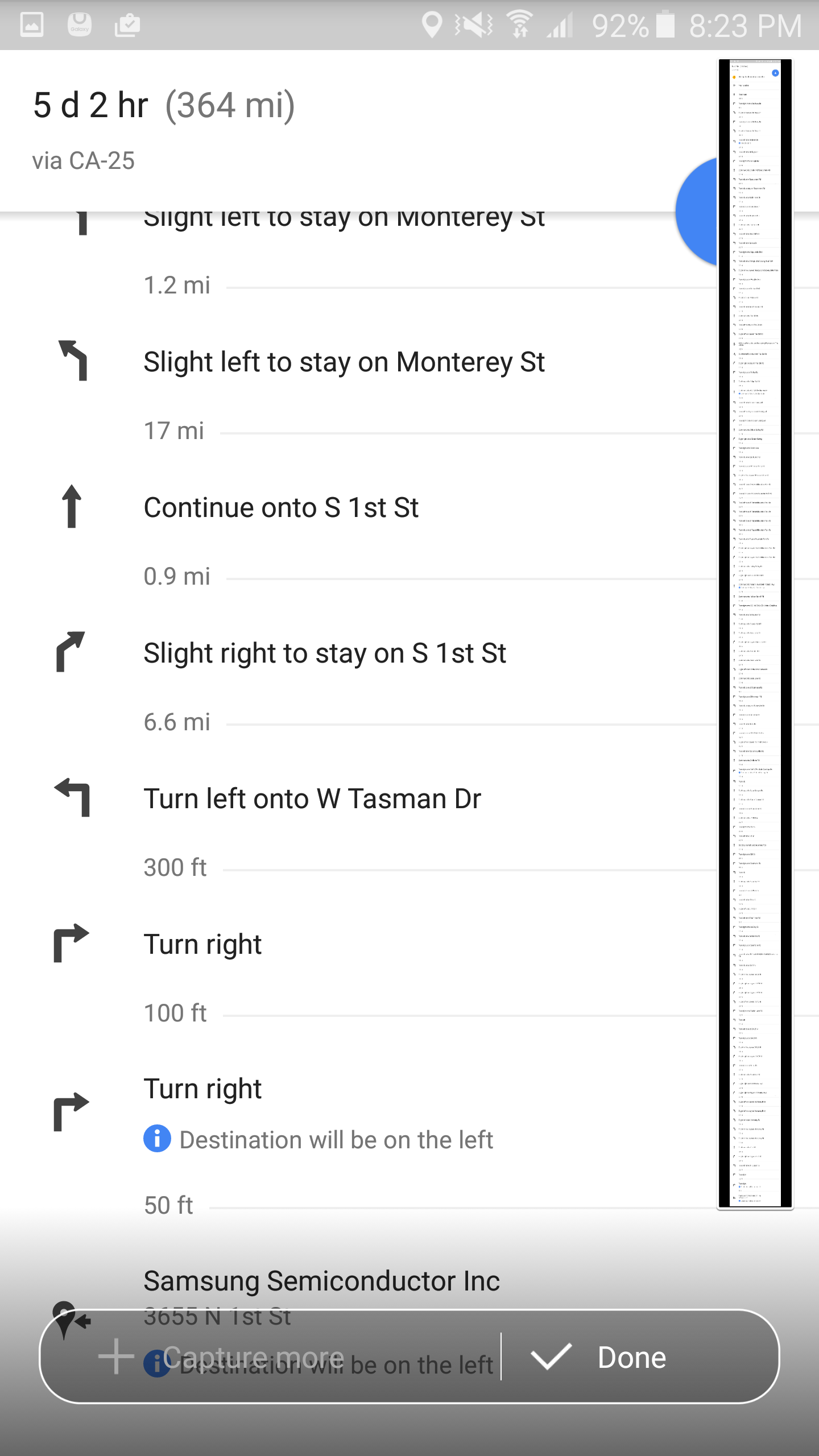This image is a screenshot taken from a mobile device and features various status icons along the top, indicating Wi-Fi connectivity, network signal strength, battery life, and the current time. The main display on the screen is a car navigation interface showing a route estimated to take five days and two hours to cover 364 miles via CA25. The navigational directions include detailed steps such as "slight left to stay on Monterey Street" and "continue on to S First Street," among others. Overlaid on the top of the screenshot is a software tool interface designed to capture the entire length of the directions as one comprehensive image displayed along the right-hand side. This overlay includes options labeled "Capture More" and "Done" for user interaction. The detailed steps of the journey are listed in a continuous sequence within the image, providing a thorough visual guide for the route.